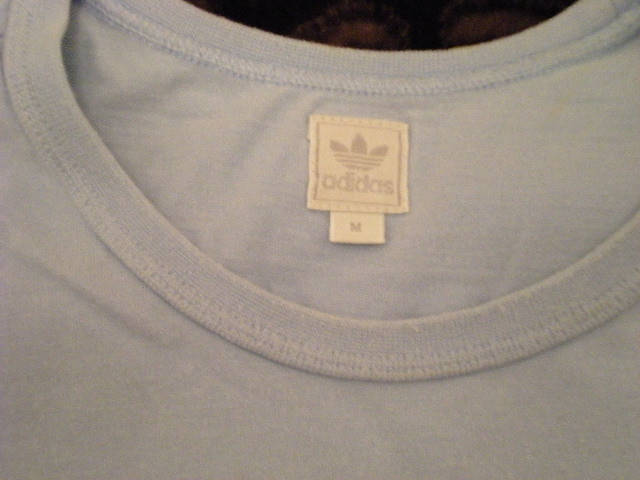The image is a detailed, close-up color photograph of the neckline of a violet Adidas t-shirt, laid flat on a wooden surface. The t-shirt is a subdued or almost faded purple, with its collar taking up most of the frame. The photograph is in landscape orientation, focusing closely on the crew neck area. The neckline features a thin hem, visibly neat with no wrinkles and is double-stitched. Prominently displayed on the inside of the back collar is a white, square Adidas tag, sewn in with white thread, showcasing the brand name "Adidas" and the three-stripe logo above it, both also in purple. Below this main tag, there is a smaller rectangular tag indicating the size "M." The background behind the collar reveals a rich, dark brown wooden surface, enhancing the focus on the shirt's details.